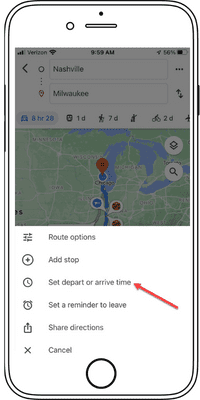The image depicts a composite view of a smartphone, showcasing both the physical exterior and a screenshot of its display. The exterior appears to be computer-generated, likely for illustrative purposes. The background is stark white.

At the top of the phone, there's a speaker area accompanied by a small black dot; to its left, there is a white circle. The phone's screen features a faintly gray GPS-like interface. From left to right along the top of the screen, the status bar displays signal strength bars, the word "Verizon," a Wi-Fi icon, the time "9:59 AM," a right-pointing arrow, "56%" indicating battery percentage, and a half-filled battery icon.

Below the status bar, two rectangular boxes labeled "Nashville" and "Milwaukee" are visible. Further down on the left, there's a highlighted oval displaying "8 hours 28 min," with a small car icon next to the number 8. Various icons representing different modes of transportation, such as walking and biking, are displayed adjacent to this time indication.

The main section of the screen shows a map centered on a location. Towards the bottom, several icons are arranged, accompanied by a prominent red arrow pointing to the option labeled "Set Depart or Arrival Time." At the very bottom of the image, there are options like "Cancel," represented with an "X," and a large circle in the center.